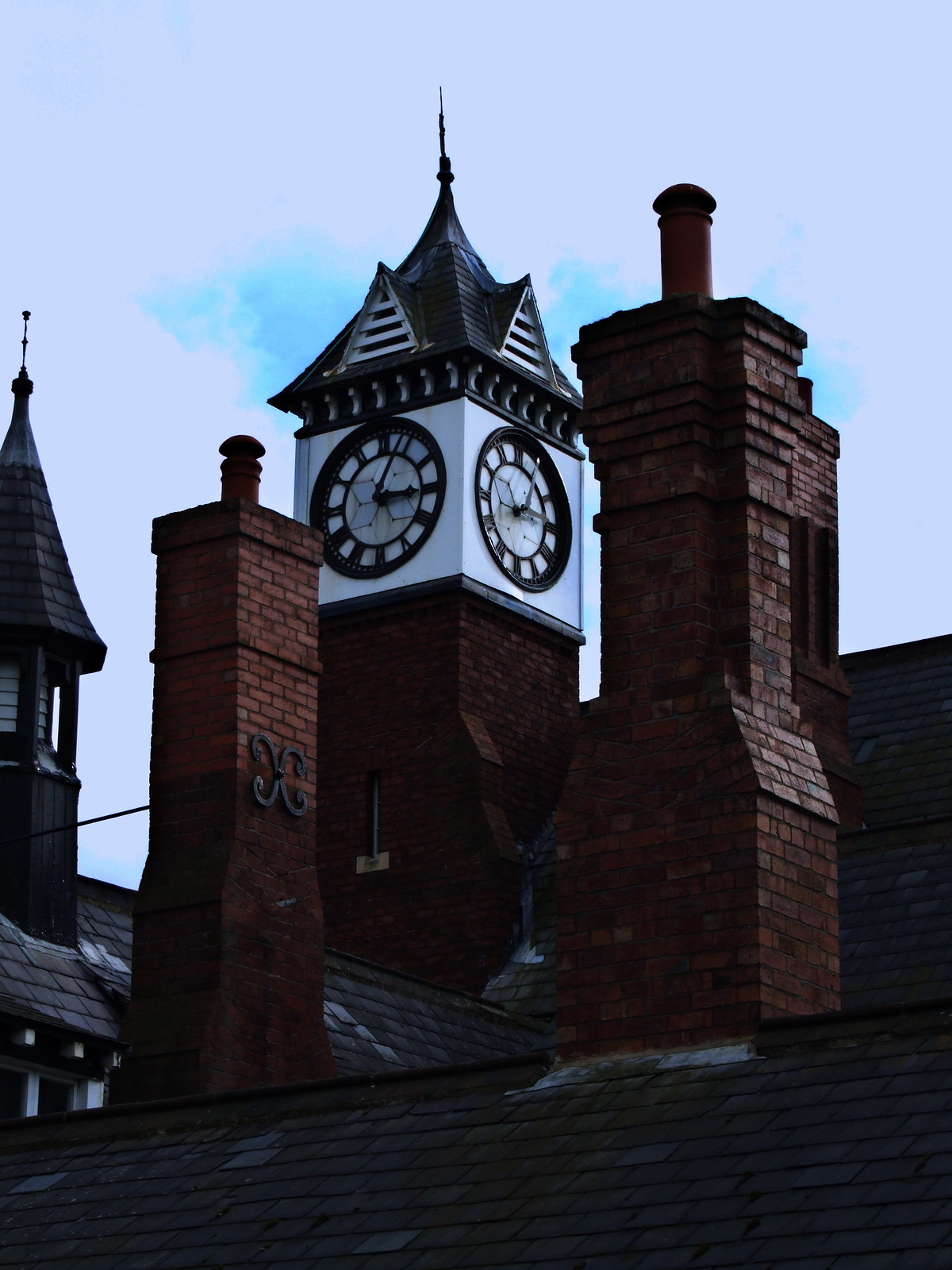The image captures an upward perspective of a striking clock tower amidst older buildings, characterized by brick chimneys and peaked rooftops. The scene has a backlit backdrop, showcasing a sky predominantly covered with white and gray clouds, although a patch of blue sky is visible around the clock tower. The buildings at the bottom of the image are enveloped in shadow, with the brick chimneys standing out in a dark red hue and the rooftops covered in gray slate. The central focus, the clock tower, rises prominently with its sturdy square structure made of dark brick. As you look higher, the clock itself is ensconced in a smooth white cube featuring two visible faces with black Roman numerals and matching black clock hands, indicating the time at approximately 3:05. Atop the clock portion, a gray, triangular-shaped roof further accentuates the tower's elegant form. To the far left of the frame, a church steeple peaks into view, and a power line cuts through the composition between the steeple and the clock tower, adding an element of urban reality to the otherwise historical scene.